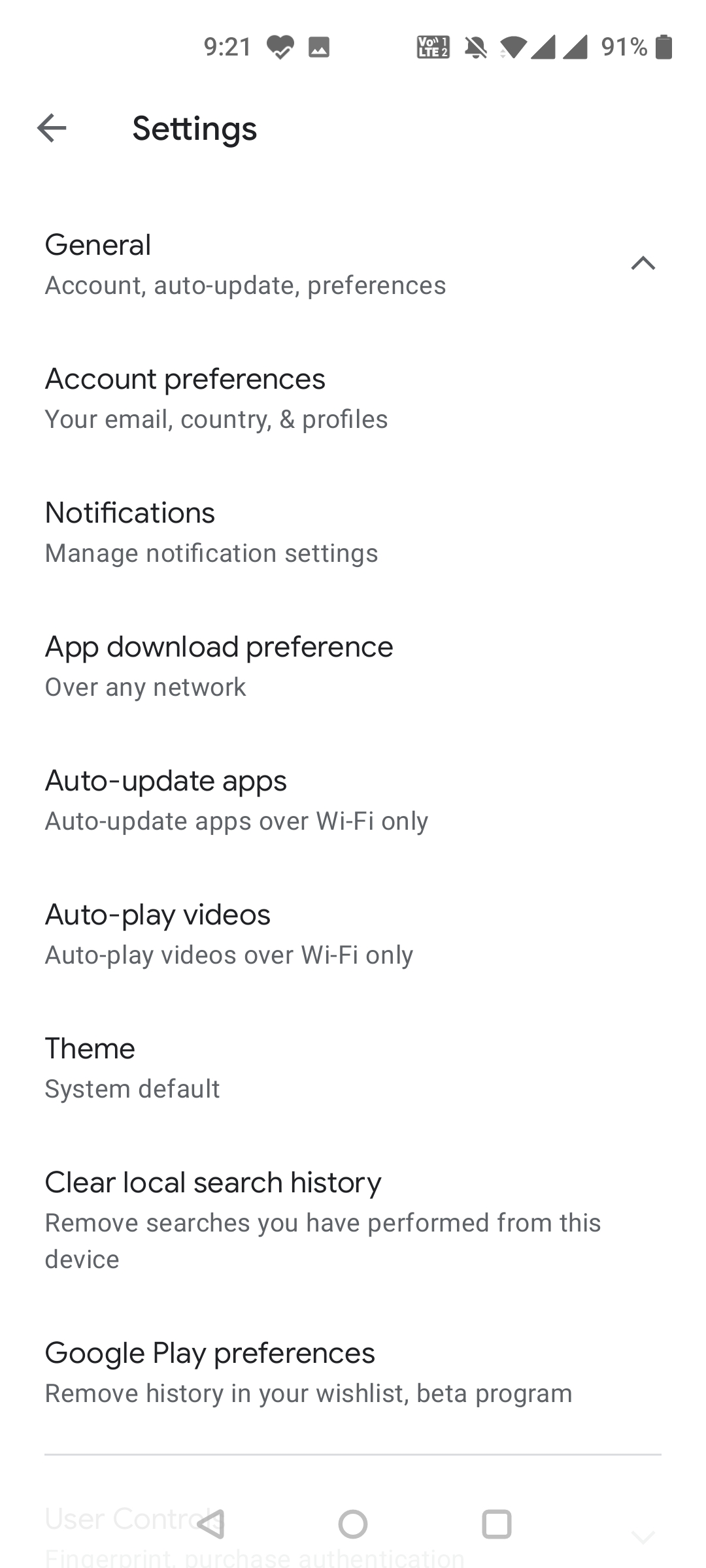The image displays a smartphone screenshot with a white background, captured at 9:21. The screenshot shows the battery at 91% and features an icon with an arrow pointing to the left below it. The screen is titled "Settings," under which several menu options are listed. These include:

- General
- Account
- Auto-Update
- Preferences

Further down, it details specific sections:

- "Account Preferences" with sub-options like "Your Email," "Country," and "Profiles."
- "Notification," specifically for "Manage Notification Settings."

Subsequent lines detail app preferences:

- "App Download Preference: Over any network"
- "Auto-Update Apps: Auto-Update Apps over Wi-Fi only"
- "Auto-Play Videos: Auto-Play Videos over Wi-Fi only"

Additionally, settings for theme and history are listed:

- "Theme: System Default"
- "Clear Local Search History: Remove searches you have performed from this device"

The final section pertains to Google Play Preferences, specifying:

- "Remove History in your wish list"
- "Beta Program"

The overall screenshot comprehensively outlines various settings and preferences available on the device.